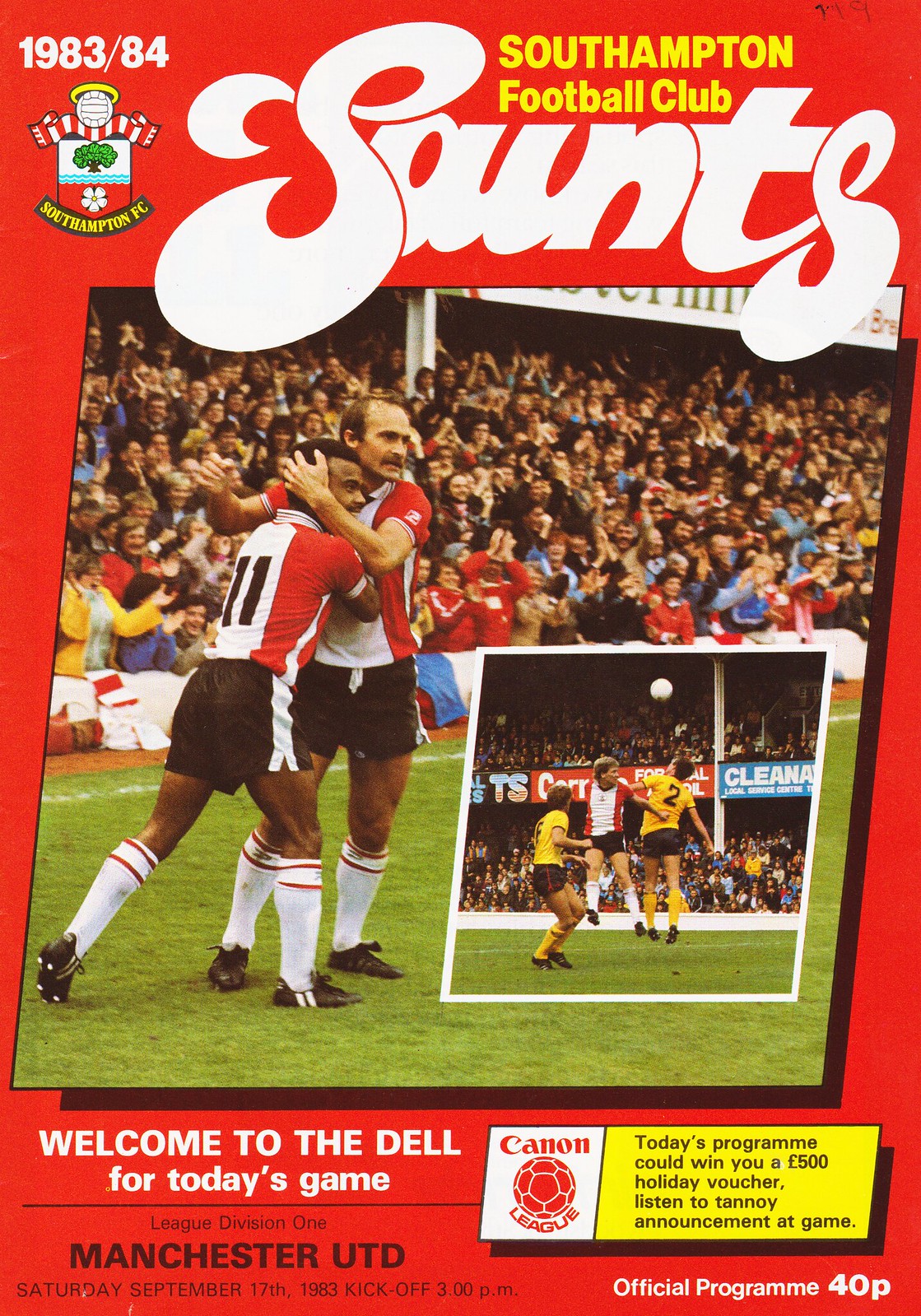The image is a vibrant and historic front page of a sports program featuring Southampton Football Club, primarily using the colors red, white, and yellow. In the top left corner, the text "1983-84" appears in white, accompanied by the Southampton FC crest. To the right, the title "Southampton Football Club" is prominently displayed in yellow letters. Below it, in a curvy and thick-lettered white font, the team name "SAUNTS" is boldly presented. 

Central to the design is a large photo depicting two soccer players embracing, with stands filled with spectators in the background. Additionally, there's an embedded image showing intense action: two players in yellow and black jerseys and another in a white jersey leaping for a header with the backdrop of a packed stadium. 

The lower left corner features the text "Canon League" alongside a soccer ball icon, with a note on an enticing opportunity to win a £500 holiday voucher by listening to announcements during the game. At the bottom of the poster, written in white letters, details about the match are provided: "Official Program, League Division One, Manchester UTD, Saturday, September 17, 1983, kick-off 3 p.m., 40 pence." Additionally, there's a welcoming message, "Welcome to the Dell for today's game."